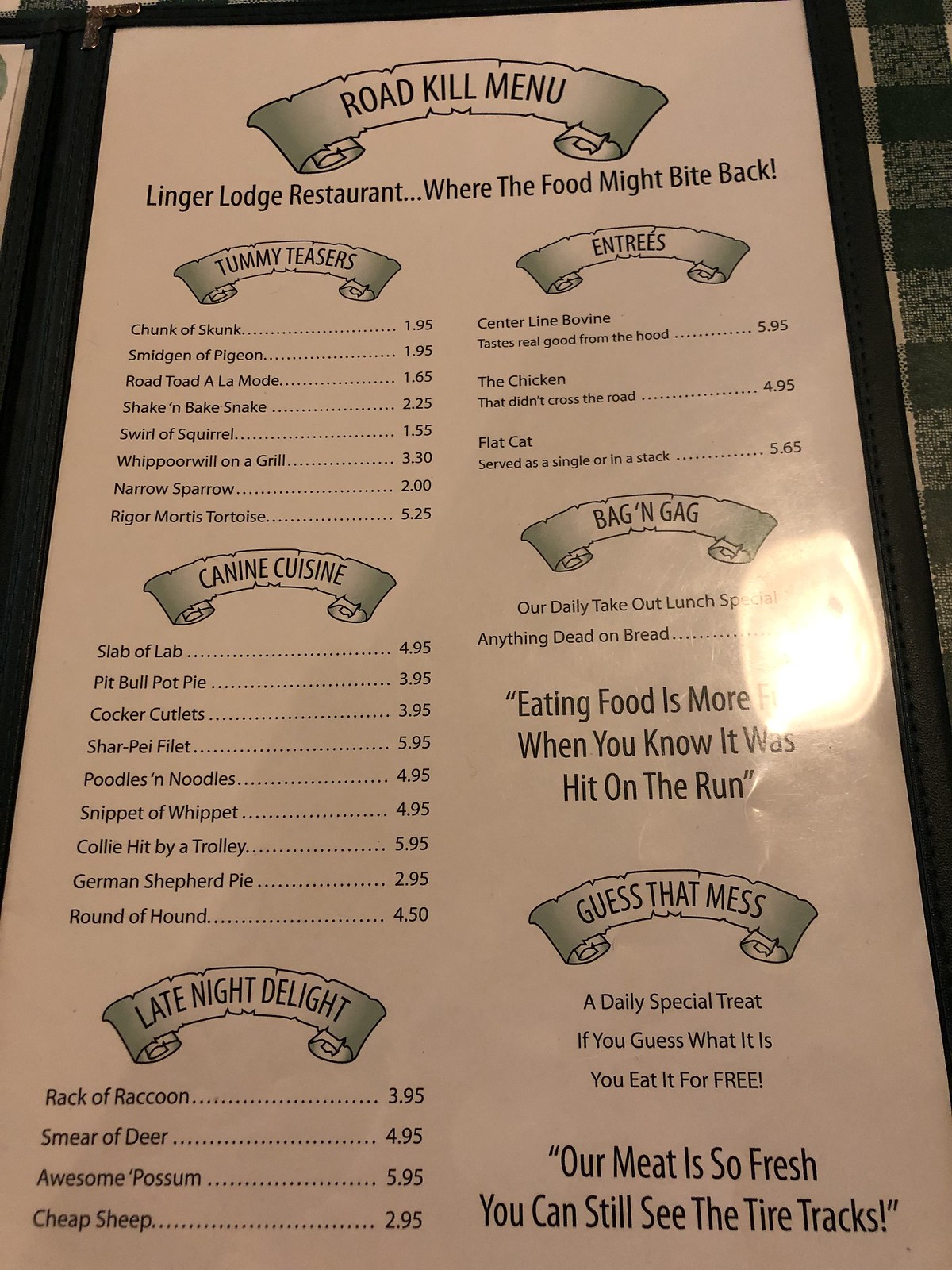This image showcases a single zoomed-in page of the "Roadkill Menu" from the Linger Lodge Restaurant, intriguingly described as "where the food might bite back." The menu page is laid out on a black, grey, and white checkered tablecloth, with a noticeable glare affecting visibility. At the top, a scroll banner proudly displays the "Roadkill Menu" title. Beneath it, in bold black font, is the restaurant’s tagline.

The menu is divided into two columns, distinguishable without any physical divider. Each column is topped by a uniquely designed banner for its subheading. The first banner reads "Tummy Teasers," and lists whimsically named dishes such as "Chunk of Skunk," "Smidgen of Pigeon," and "Road Toad à la Mode," each accompanied by prices. Another banner titled "Canine Cuisine" introduces additional dishes and includes a special section for "Late Night Delights."

The second set of columns features main courses under banners such as "Entrees," "Bag and Gag," and "Guess That Mess." The humorously morbid theme continues with creatively named dishes. 

At the bottom right of the menu is a boulder-shaped logo with the quirky slogan, “Our meat is so fresh you can still see the tire tracks," presented within quotation marks. Additionally, a larger font at the bottom encourages a playful perspective on the dining experience with the phrase “Eating food is more fun when you know it was hit on the run.”